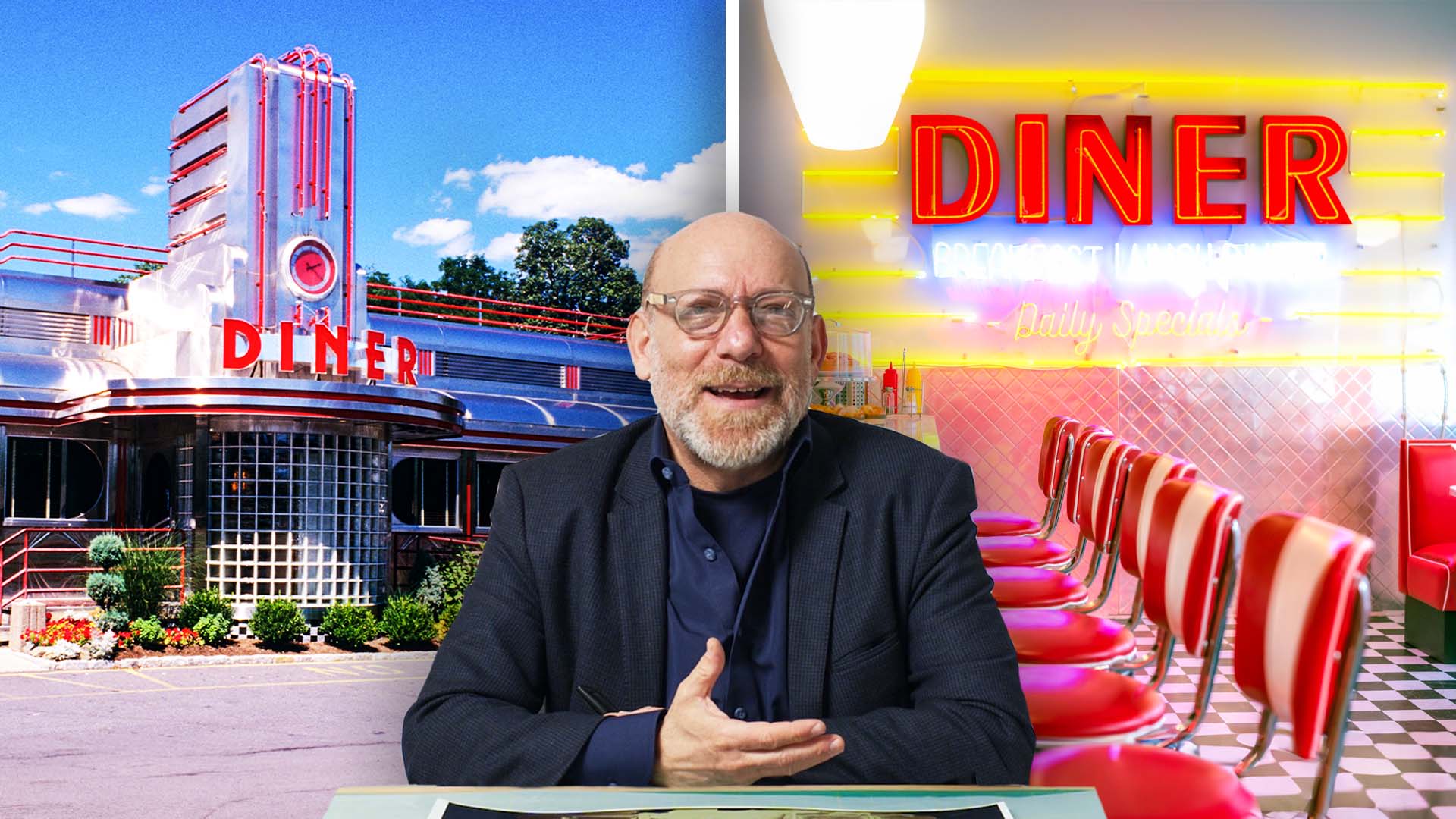The image is a wide, rectangular, seemingly Photoshopped composition featuring two juxtaposed scenes of a diner and an older man. The left side of the image showcases an outdoor diner sign with a gradient roof, transitioning from white to green to blue, topped by a light blue sky with faint clouds. The bright red neon letters spell "diner" above a band of horizontal red diamond patterns, beneath which a window with drawn blinds is visible. On the right side, an indoor scene is depicted with a black and white checkered floor and two rows of red booths, each accompanied by a white table.

Centrally overlapping these scenes is an elderly man with a bald head, gray beard, and glasses, dressed in a navy blue collared shirt and matching suit jacket. He appears to be either sitting or standing in front of a small table or podium, with his mouth open as if speaking. The juxtaposition and visual incongruity of the man's position suggest he may have been digitally inserted into the diner setting. The diner itself has an old-fashioned aesthetic, and no other people are visible in the image.